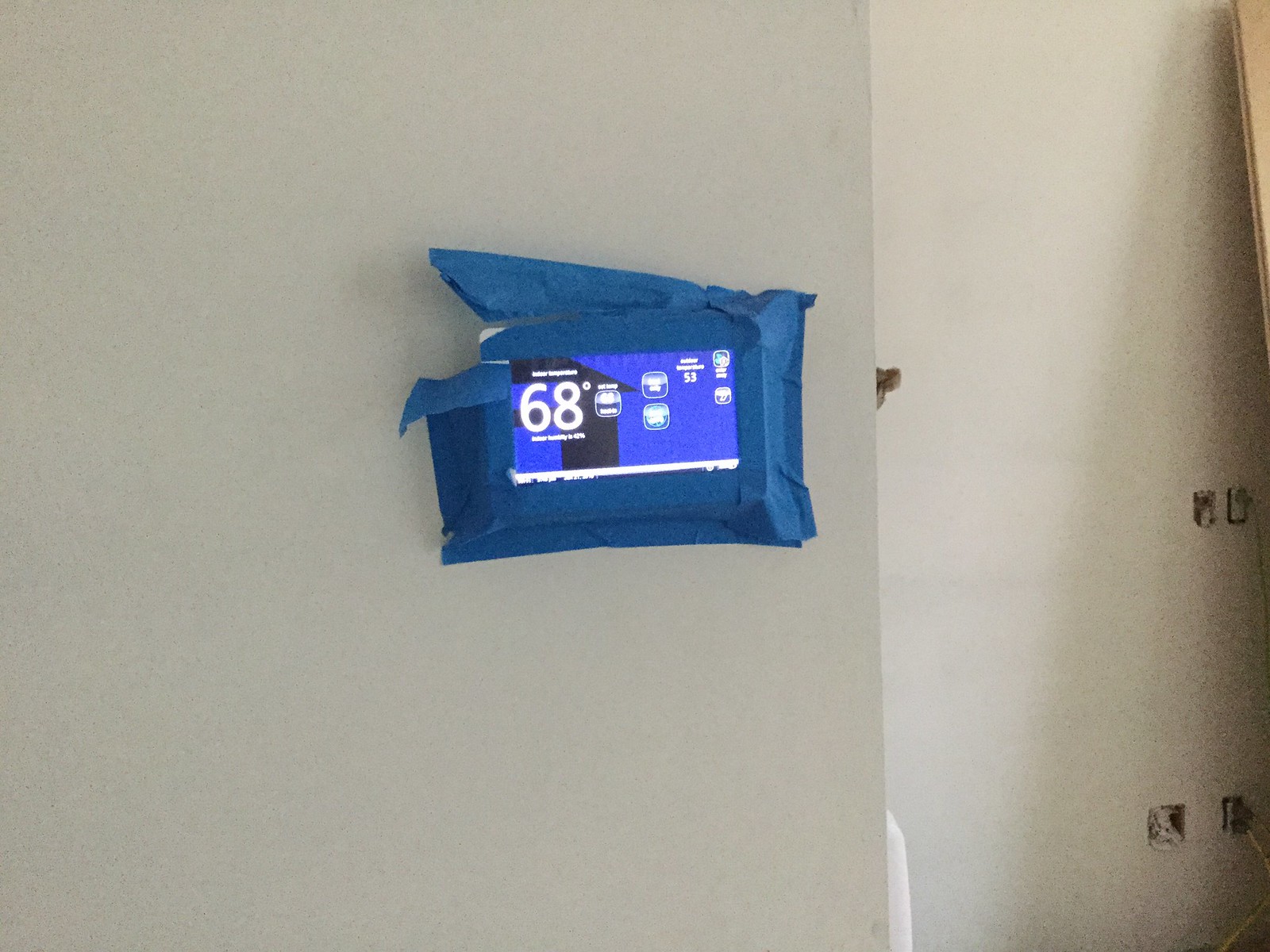The image showcases a commercial thermostat displaying a temperature of 68 degrees, with an external temperature indication of 53 degrees. The device's interface is surrounded by blue painter's tape, suggesting ongoing preparations for wall painting. The thermostat's screen features various symbols, including a royal blue background with a black house icon. Electrical outlet plates are removed, further indicating painting activity. In the upper right-hand corner, another wall painted in a medium tan color is partially visible, along with a hanger aligned almost level with the thermostat. This creates a sense of an in-progress renovation or maintenance work in the room.